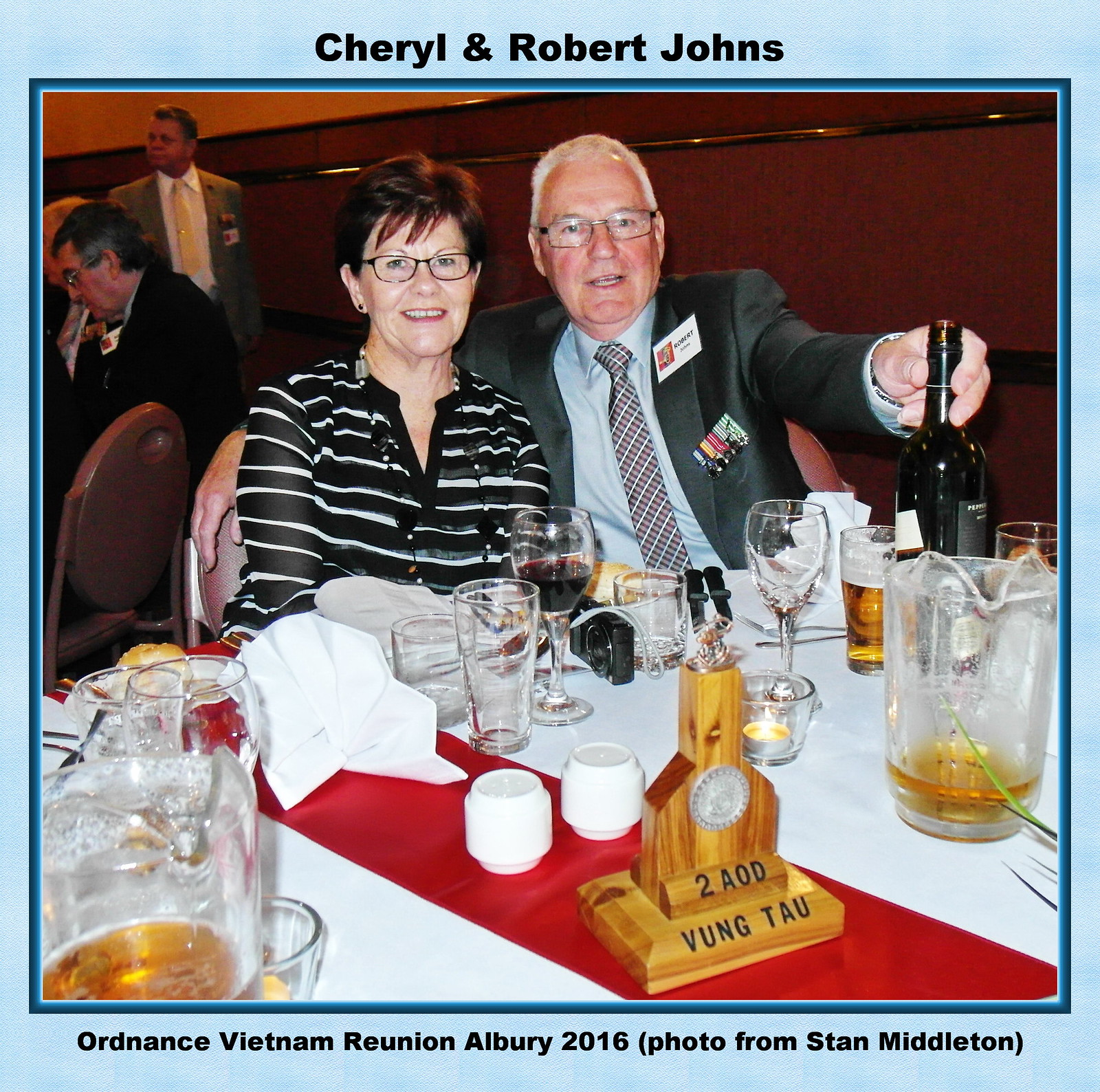This photograph captures a moment from the Ordnance Vietnam Reunion in Albury, 2016, as noted by the black text at the top and bottom of the light blue bordered image reading "Cheryl and Robert Johns" and "Ordnance Vietnam Reunion Albury 2016 (photo from Stan Middleton)." Centrally positioned are Cheryl and Robert Johns, an older couple enjoying what appears to be a lively dinner party. Cheryl, seated to the left, wears a black and white horizontally striped shirt, glasses, and has short brownish-red hair, suggesting she is in her late 50s or 60s. To her right is Robert, an older man with white hair, black glasses, clad in a black sports jacket, light blue shirt, and a multicolored tie. His name tag reads "Robert," and his left hand rests on a bottle of wine. The table in front of them, covered in a red and white tablecloth, hosts several glasses of beer and other dinnerware. A wooden centerpiece, bearing the inscription "2AOD Vung Tau," adds a personal touch to the reunion's ambiance. In the background, other attendees, also dressed in suits, are seen engaging in conversation and enjoying the event.